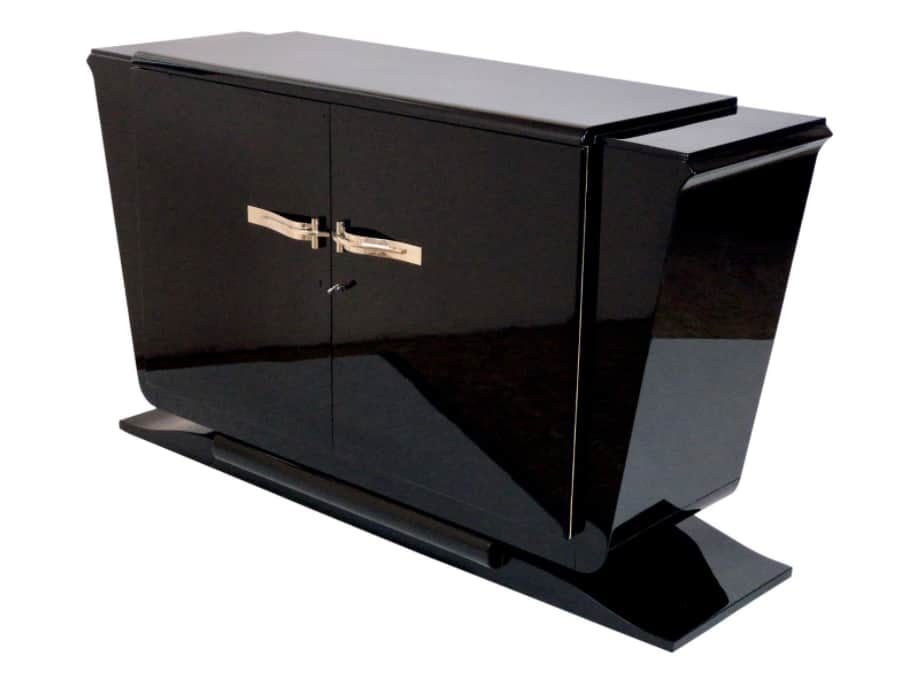This image showcases a sleek, glossy black cabinet set against an entirely white background. Captured from a front-facing angle with a slight view of the left corner, the cabinet features two vertical, rectangular doors, each adorned with a reflective gold handle. The door on the right appears to have a key inserted into a lock. The cabinet's lustrous surface highlights reflections, particularly noticeable on the top and left side.

The cabinet sits atop a flat black base that extends slightly outward and curves down at the edges. The cabinet's side panels angle up and outward, giving it a flared appearance as they rise. The top of the cabinet is flat and practical for resting items. The overall design is both modern and functional, emphasizing its shiny, black finish and graceful contours.